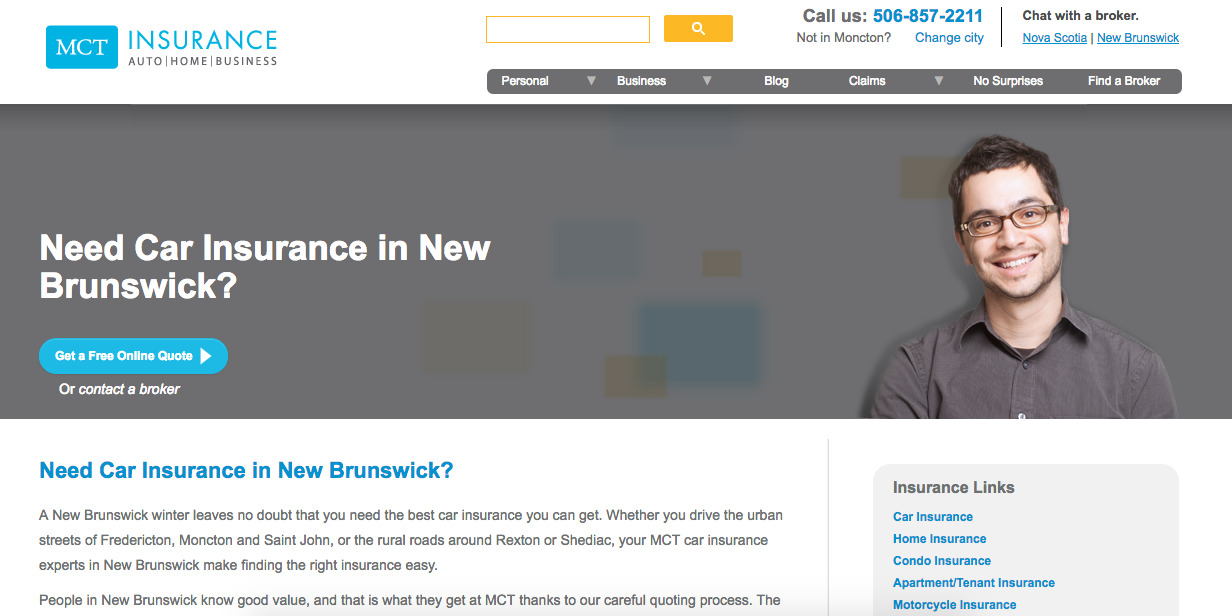This is a screenshot of an insurance agency's website. In the upper left-hand corner, there is a light blue rectangle featuring the initials "MCT" in bold letters. Adjacent to this logo, the text "Insurance Auto Home Business" is displayed prominently. Positioned at the center of the page's top section is a small, yellow search bar. Beneath this search bar are several dropdown menus labeled "Personal," "Business," "Blog," "Claims," "No Surprises," and "Find a Broker." A telephone number in blue font is conspicuously placed at the top of the page for easy customer access.

Dominating the central portion of the page is a large banner with a gray background and white text that reads, "Need Car Insurance in New Brunswick?" Positioned below this message is a blue button with white text encouraging visitors to "Get a Free Online Quote." To the right of the button, there is an image of a smiling man wearing glasses and a button-down shirt, adding a personable touch to the site.

Further down the page, set against a white background, is an additional section of content with blue and dark gray text. The heading reiterates the key message: "Need Car Insurance in New Brunswick?" reinforcing the banner above.